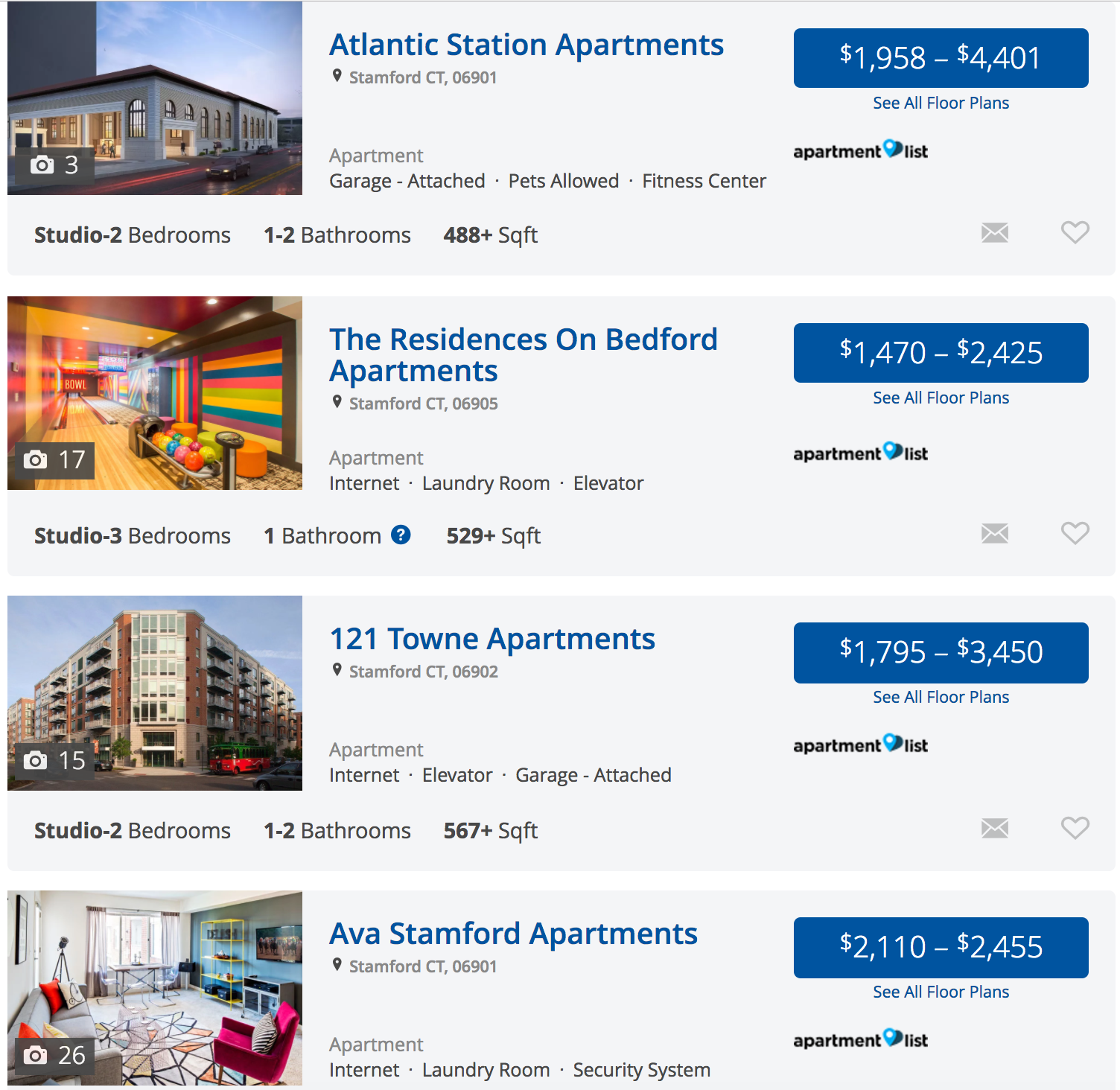Atlantic Station Apartments in Stamford, CT 06901, offer a range of rental options priced between $1,958 and $4,401. Floor plans are available for studios to two-bedroom units with one to two bathrooms, covering 488 square feet (SQFT). 

Additionally, The Residences on Bedford in Stamford, CT 06905, provide apartments ranging from $1,470 to $2,425. These units include studios to three bedrooms with one bathroom, starting at 529 square feet (SQFT). 

Lastly, the townhomes in Stamford, CT 06902 are available for rent from $1,795 to $3,450. Options include studios to two-bedroom units with one or two bathrooms, starting at 567 square feet (SQFT).